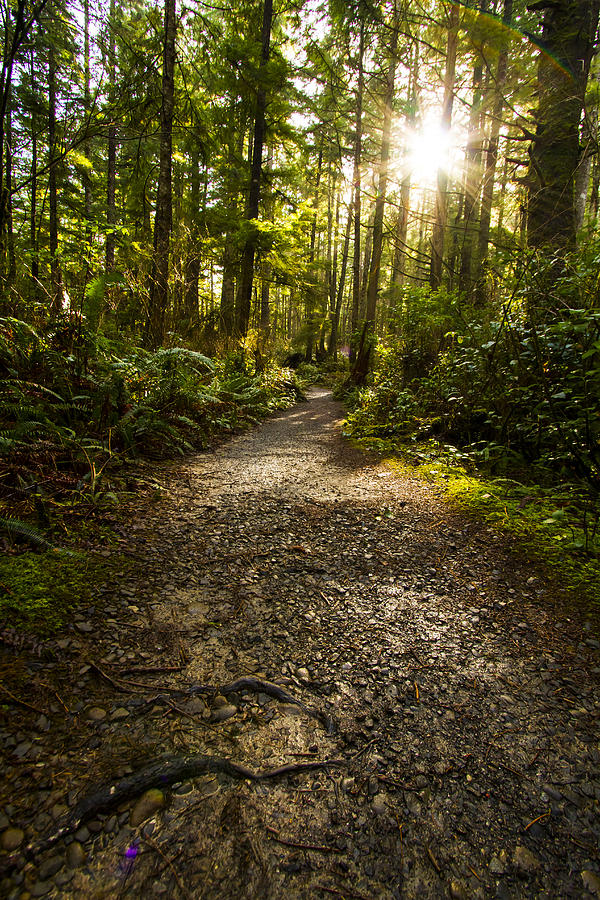The photograph captures a serene forest scene with a dirt path meandering through tall, slender conifer trees, flanked by shorter shrubs and herbaceous plants. The trees, closely spaced and uniform in height, suggest they grew around the same time, adding to the collective tranquility of the forest. Dappled sunlight filters through the foliage, creating a warm, golden glow that bathes the entire scene, particularly concentrated in the upper right corner of the image. This sunlight reaches the forest floor in scattered patches, enhancing the earthy browns of the dirt path and the tree trunks. The path is mostly clear with a few visible twigs, stones, and tree roots, adding texture to the scene. In the lower left corner, a small purple object, possibly litter, is subtly noticeable. The overall palette of the image is dominated by natural greens, browns, and golden yellows, invoking a sense of peaceful seclusion and natural beauty. The enclosing greenery along the sides of the path contributes to the intimate, almost enclosed atmosphere of this tranquil forest setting.